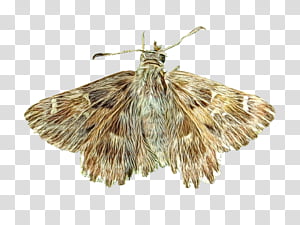The image depicts a moth on a gray and white checkered background, commonly used for transparency in image editing programs like Photoshop and GIMP. The moth's condition appears worn, with scraggly, damaged wings and bent antennae. The left antenna is notably bent almost horizontally with a black tip, while the right antenna is forward and diagonally placed but similarly damaged. The moth is mostly brown with a mix of beige and tan, featuring darker spots more concentrated on the left wing than the right. Its wings have a subtle pattern of polka dots, with some dots appearing dark brown, orange, or blending into the brown and beige mix. The body of the moth is partially light brown and partially white, with its head slightly tilted, revealing its right eye but obscuring the left. The moth's appearance is reminiscent of a drawing due to the low resolution of the image, and despite the somewhat pixelated and damaged quality, it's clear enough to distinguish these intricate details.